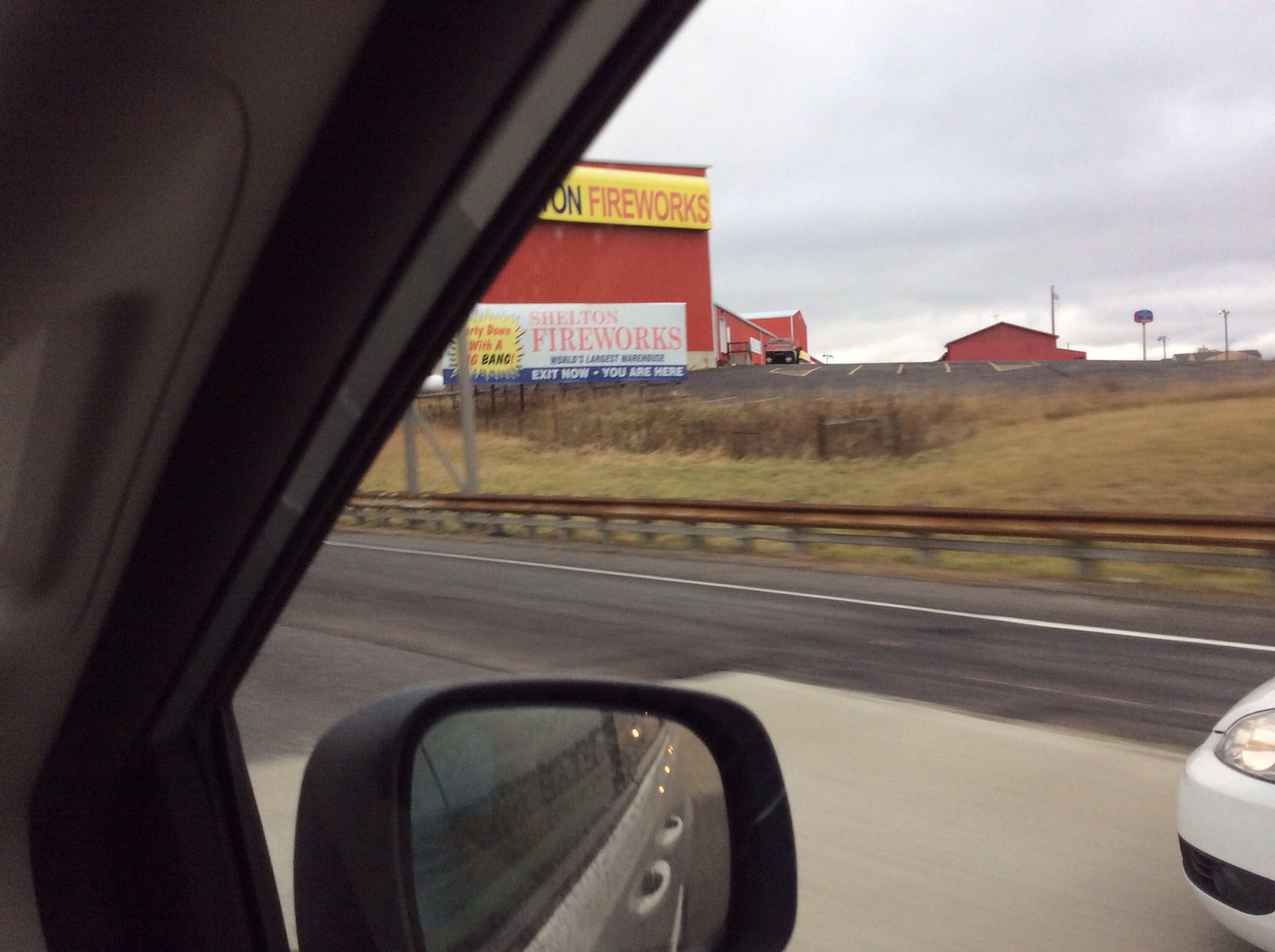This photograph, captured from the passenger seat of a moving vehicle, displays a detailed scene from a journey along an asphalt road. The photo includes the outline of the silver, four-door car and its side mirror. A passenger, potentially a woman, is visible with both hands gripping the camera to take the shot. The road scene includes the front left portion of a white vehicle in the adjacent lane, headlights on, and a rusty guardrail lining the road. Beyond the guardrail stretches a field of brown grass, hosting a prominently positioned billboard. This billboard, mounted unusually low to the ground, features a vivid red background with a yellow banner at the top. The word "Fireworks" is boldly displayed in red, and the bottom of the billboard is sectioned into two banners: a white one that reads "Shelton Fireworks" and a blue one proclaiming "Exit Now, You Are Here." The photograph captures a fleeting yet vivid moment of travel.